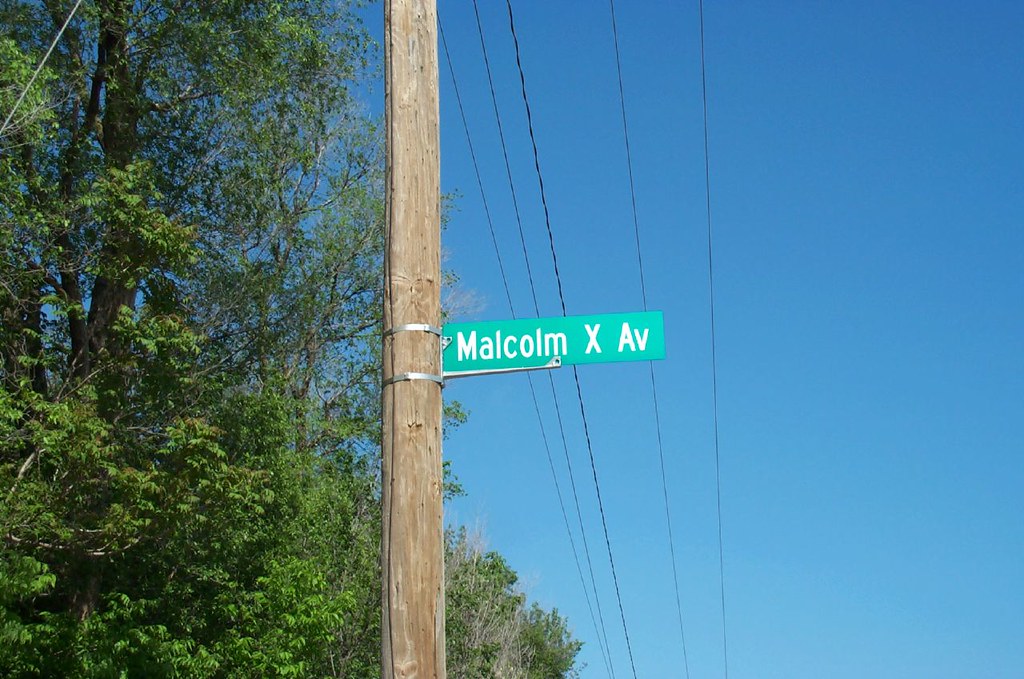In this image, a prominent street sign is affixed to a light brown, wooden telephone pole, visible from its base to its top. The pole features two silver rings around its center, securing the sign in place. The sign itself is horizontal, rectangular, and light green with the text "Malcolm X Ave" displayed in white letters. To the left of the pole, a lush backdrop of green trees fills the scene, while the right side reveals five telephone wires stretching behind the sign. The sky above is a clear, vivid blue, providing a bright and contrasting background.